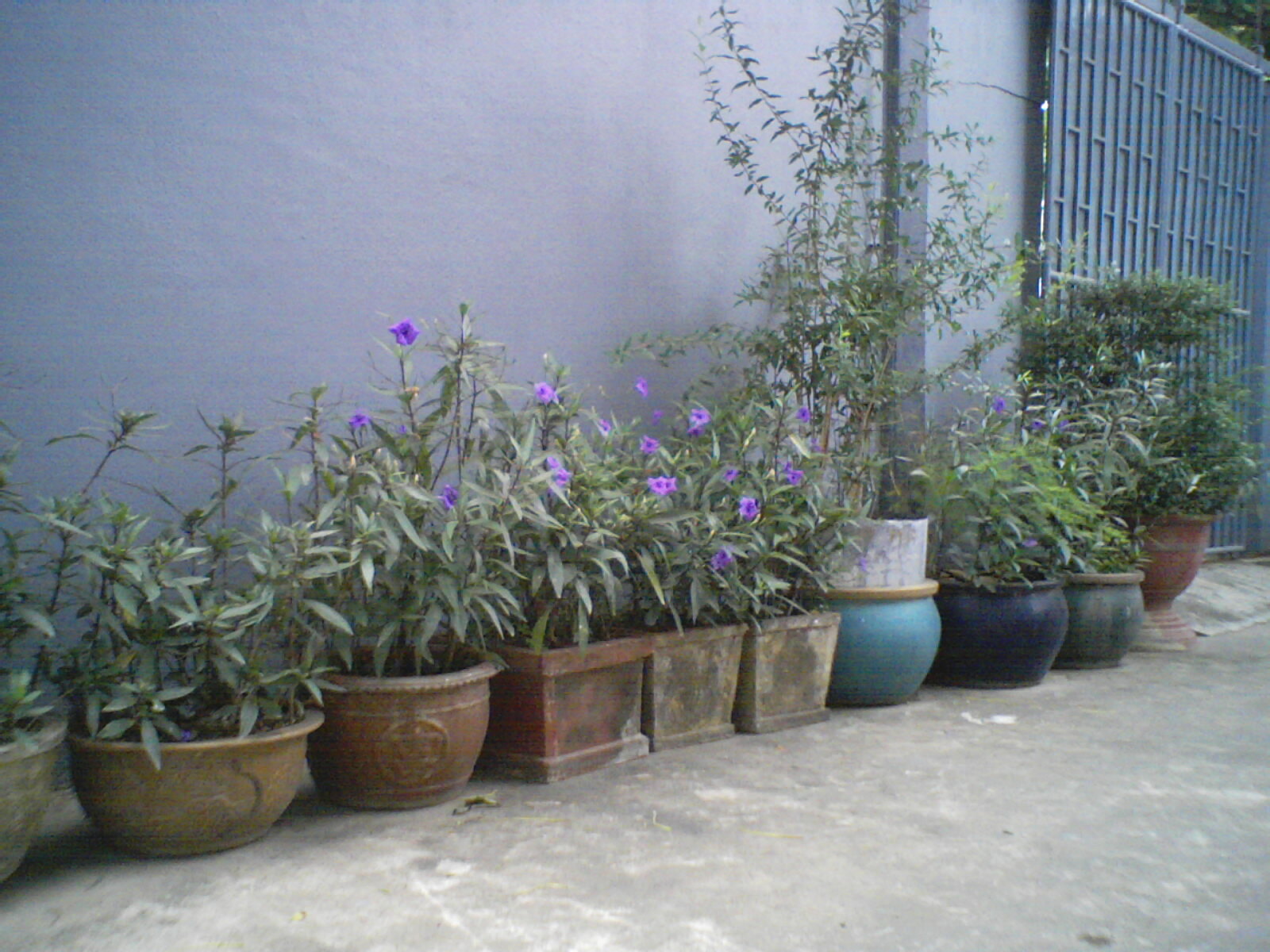This photograph captures a vibrant outdoor scene featuring a series of ten ceramic planters lined up on a concrete sidewalk against a blue stucco wall. On the right side of the image, a gray metal gate complements the urban setting. Each pot varies in shape and color, ranging from natural terracotta and black to blue, tan, and brown, with some featuring decorative gold rims. The planters house a diverse array of plants; six of them boast tall, blooming purple flowers, while others consist of lush green foliage and shrubs. One notable planter near the gate contains a gangly young tree, adding to the charming, botanical display.